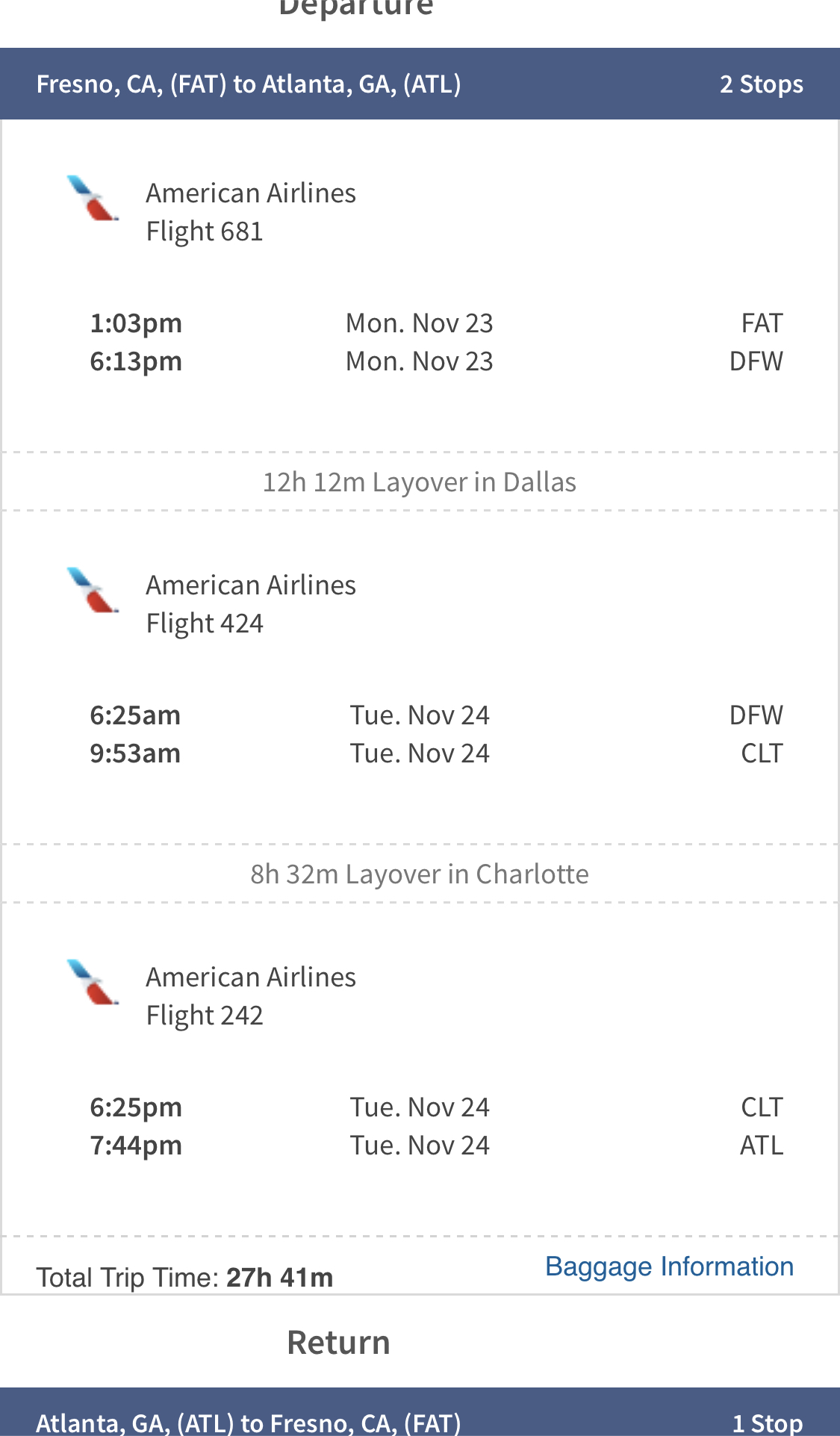The image is a detailed screenshot of a flight itinerary, most likely taken from a travel booking page. The itinerary belongs to American Airlines and features the airline's emblem, a bird with blue and red wings. The traveler's journey begins with a departure from Fresno, California (FAT), heading to Atlanta, Georgia (ATL), with a total of two stops.

1. **First Leg**:  
   - **Flight**: American Airlines Flight 661  
   - **Departure**: 1:03 PM on Monday, November 23rd from Fresno (FAT)
   - **Arrival**: 6:13 PM on Monday, November 23rd at Dallas/Fort Worth (DFW)  
   - **Layover**: 12 hours and 12 minutes in Dallas   

2. **Second Leg**:  
   - **Flight**: American Airlines Flight 424  
   - **Departure**: 6:25 AM on Tuesday, November 24th from Dallas/Fort Worth (DFW)  
   - **Arrival**: 9:53 AM on Tuesday, November 24th at Charlotte (CLT)  
   - **Layover**: 8 hours and 32 minutes in Charlotte  

3. **Third Leg**:  
   - **Flight**: American Airlines Flight 242  
   - **Departure**: 5:25 PM on Tuesday, November 24th from Charlotte (CLT)  
   - **Arrival**: 7:44 PM on Tuesday, November 24th at Atlanta (ATL)

The total trip time amounts to 27 hours and 41 minutes. Below these details, there is a section for baggage information and a partially visible return itinerary, indicating a return trip from Atlanta, Georgia to Fresno, California with one stop, but the specific details are cut off at the bottom of the image.